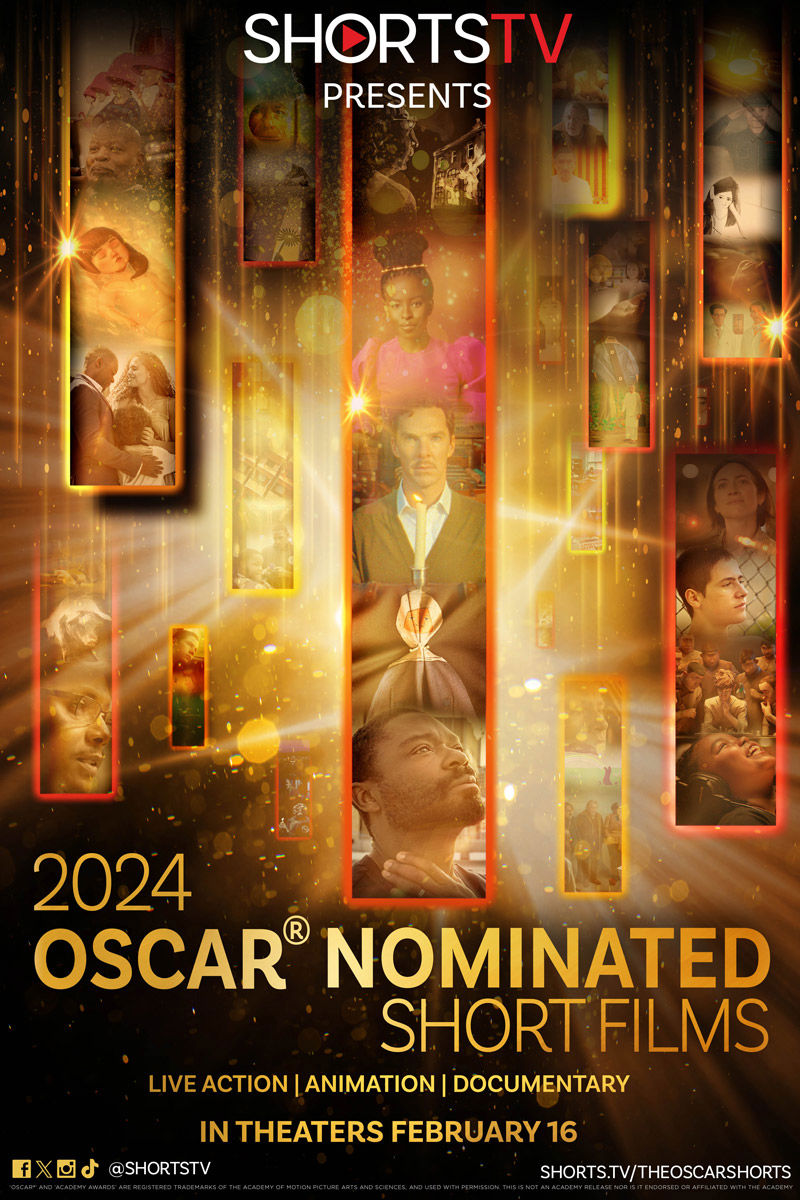This is an advertisement poster for the 2024 Oscar-nominated short films, presented by Shorts TV. At the top, "Shorts TV presents" is prominently displayed with "Shorts" in large white letters and "TV" in red. The central part of the poster is filled with numerous tall rectangular images featuring stills from the nominated films, in a layout that evokes the look of film strips suspended in space. The background is dark brown with a visually dynamic array of gold, yellow, and red hues, creating a busy and bright atmosphere accentuated by reflections and linear paths of strobing light.

Towards the bottom in gold lettering, it reads "2024 Oscar-nominated short films" with additional information below it: "Live Action, Animation, Documentary" and "In Theaters February 16th." On the bottom right, there's the website "shorts.tv/theoscarshorts" and, on the left, the logos of various social media and music platforms such as Facebook, X (formerly Twitter), and Google Music, along with the handle "@ShortsTV."